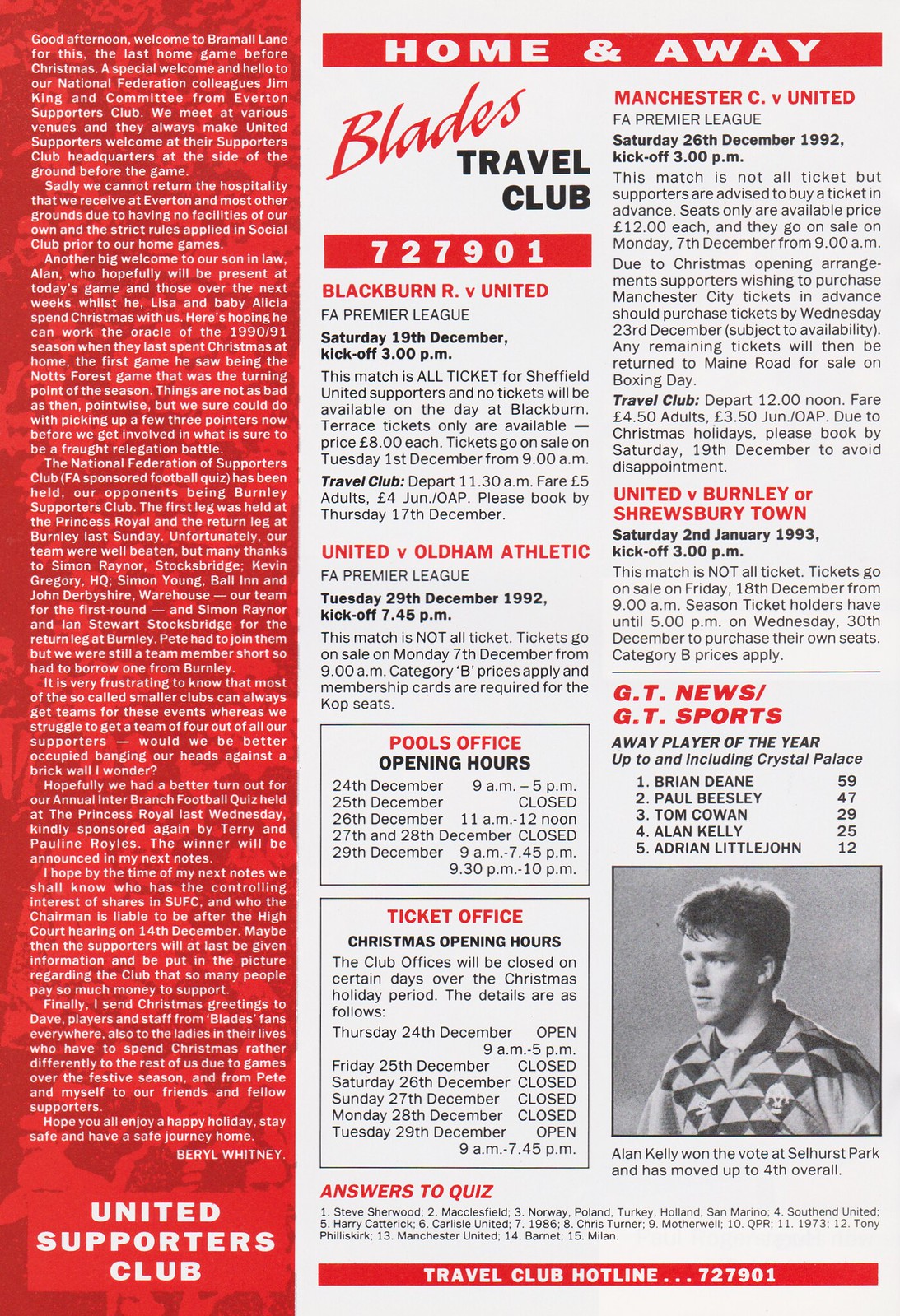The image is a scanned page from a football (soccer) magazine or pamphlet, featuring the United Supporters Club. The left side of the page showcases a vertical red rectangle with white text at the bottom reading "United Supporters Club." The rest of the page is predominantly white, with a red rectangular header at the top stating "Home and Away Blades Travel Club" and the number "727901." Below this header, the page details various upcoming football matches including "Blackburn Rovers vs. United" on Saturday, December 19th at 3 p.m., and "United vs. Oldham Athletic" on Tuesday, December 29th, 1992, at 7:45 p.m., among others. It also lists new Christmas opening hours for the Poole's Office and Ticket Office. In the bottom right corner, there is a black-and-white photograph of a man in a soccer uniform looking to the left, captioned "Alan Kelly won the vote at Selhurst Park and has moved up to fourth overall."